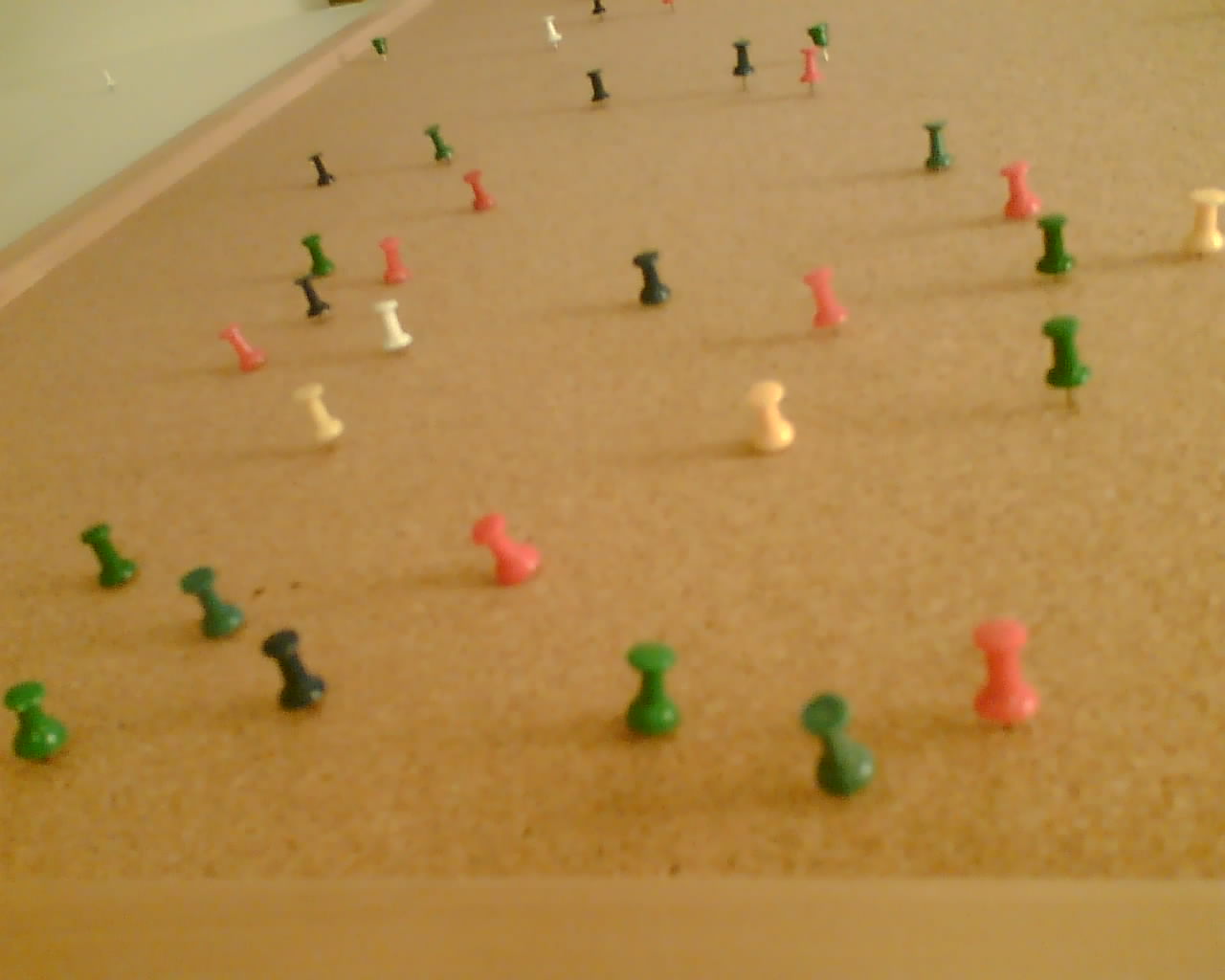This image features a close-up of a tan cork bulletin board with a wooden frame. The board is covered with a variety of colorful plastic pushpins, including green, pink, yellow, white, black, and even some dark blue ones. The pushpins are scattered randomly across the board with no particular pattern—some are clustered while others are more spaced out. There are no notes or notifications pinned to the board at the moment. The background visible behind the board appears to be a tan or beige wall, and there's a light green area noticeable in the upper left corner of the image. The scene conveys a somewhat haphazard array of pushpins, suggesting they have been previously used and then placed back on the board in a random order.